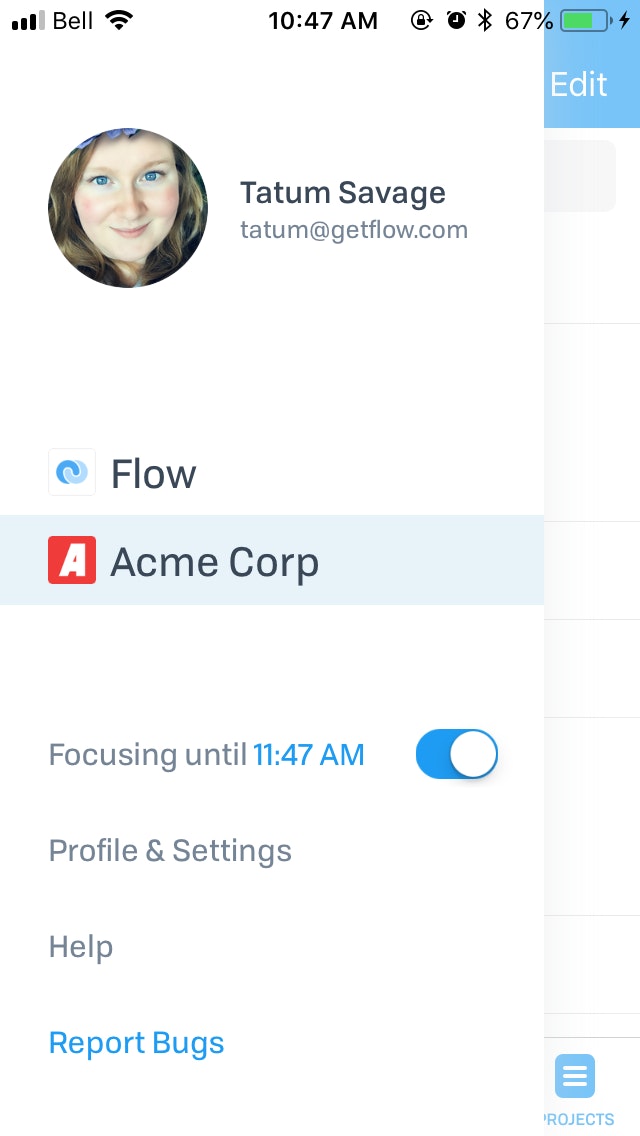The image is a screenshot from a cell phone, with dimensions approximately two and a half times as tall as it is wide. In the upper left corner, the wireless signal icon shows three out of four bars, next to the label "Bell," with a fully filled cell signal icon beside it. Centered at the top, the time is displayed as 10:47 a.m. To the upper right are several icons, including a battery icon indicating a 67% charge, filled in green, with a lightning bolt symbolizing that the phone is currently charging.

Below this status bar, the screenshot appears to be within an app. At the top, there is a profile picture of a young Caucasian woman smiling, identified as "Tatum Savage," with her email, Tatum@getflow.com, displayed underneath. An icon with two swirled shades of blue featuring the word "flow" is present below her email.

Following this, there's a red box with a white "A," labeled "Acme Corp." Below this, a line of text reads "Focusing till 11:47 a.m.," with a toggle switch to the right which is turned on. Further down are options labeled "Profile and settings," "Help," and, in light blue, "Report bugs."